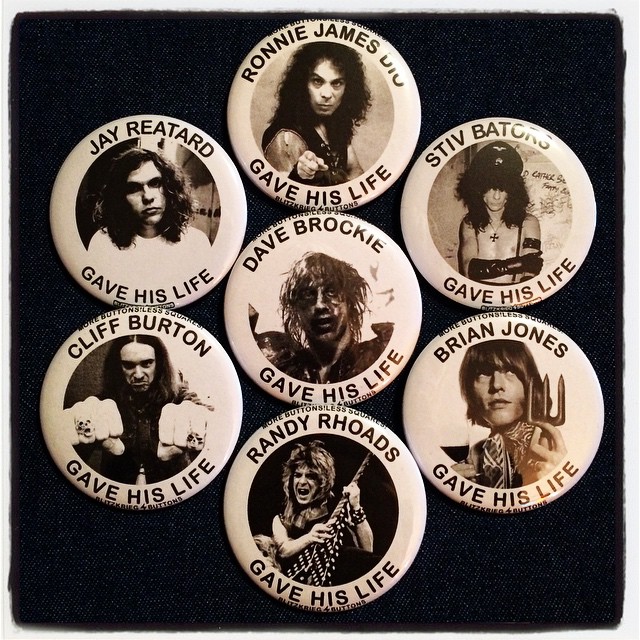The photograph features seven commemorative button badges arranged on a dark fabric, which could be either black or dark blue jean material, forming a circular pattern. Each badge prominently displays a black and white image of a person along with their name above and the phrase "Gives His Life" below. 

At the top of the circle is a badge with the name "Ronnie James Dio." To the upper left is "Jay Reatard," depicted as a man with long wavy hair wearing a white shirt. The badge on the upper right features the name "Steve Baders." In the center of the circle, the badge reads "Dave Brockie." Below Dave Brockie, there is another badge showing a man holding a guitar with the name "Randy Rhoads." At the bottom left, beneath Jay Reatard, is "Cliff Burton." Finally, in the bottom right corner is a badge honoring "Brian Jones." 

Each button is a tribute to these individuals, emphasizing their contributions and sacrifices.